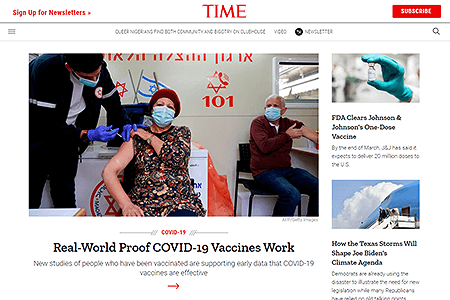This image captures a screenshot of the TIME website's homepage. At the top center, the iconic "TIME" logo is prominently displayed in all capital letters, featuring its traditional red font. To the left of the logo, there is a "Sign Up for Newsletters" prompt also in red font, accompanied by an adjacent arrow or dot. On the far right, a red "Subscribe" button is visible within a rectangular box, delineated by an underscoring line.

To the left of the central logo, a hamburger menu icon is present. Some indistinct text, likely in English, appears around the middle, featuring a black dot nearby. Positioned all the way to the right is a magnifying glass icon, indicating a search function. Directly below this top navigation bar is a thin dividing line.

The main content area of the page features a prominent media image of a woman receiving a vaccination. The woman has her right shoulder exposed, wears a mask, and dons a headscarf and a long-sleeve dress. A medical professional is administering a shot into her shoulder. To the right of the woman, another masked individual is seen adjusting his garment. The image is headlined with "Real World Proof COVID-19 Vaccine Works," and includes a "101" label alongside a Star of David symbol in the background.

Adjacent to this main feature, there are two additional articles on the right-hand side, each accompanied by their own images.